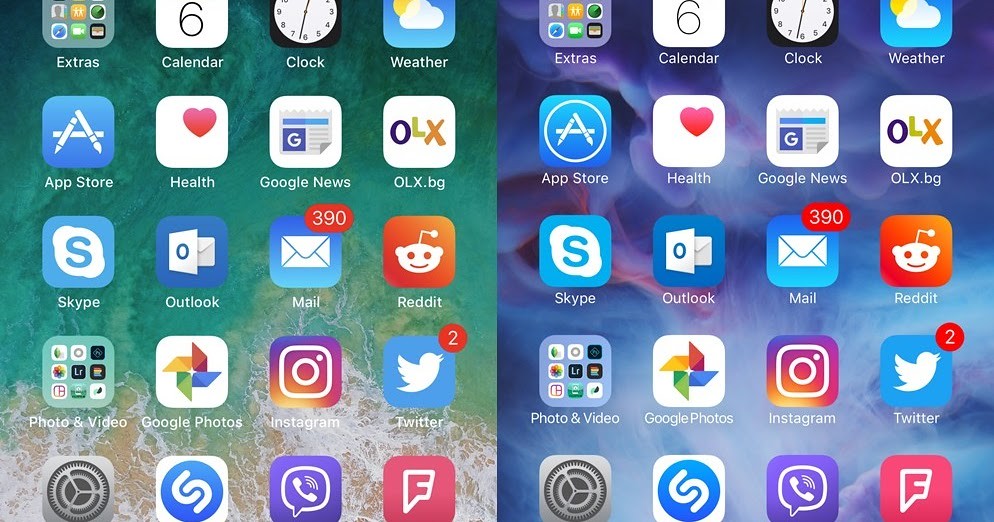The image consists of two side-by-side screenshots of an iPhone home screen. The set of apps and their arrangement are identical in both screenshots. The apps visible include an extras folder, Calendar, Clock, Weather, App Store, Health, Google News, OLX.bg, Skype, Outlook, Mail (showing 390 unread emails), Reddit, a Photos and Videos folder, Google Photos, Instagram, Twitter (with 2 notifications), a Settings folder, another Skype icon, a messaging app, and Foursquare.

The main difference between the two screenshots is the wallpaper. The screenshot on the left features a beach-themed wallpaper depicting a serene turquoise ocean meeting sandy shores, with white frothy waves caressing the beach. The screenshot on the right, however, showcases an abstract wallpaper with pink and white hues resembling swirling smoke or flames. 

Both screens are filled with the same apps, maintaining the same notifications and layout.